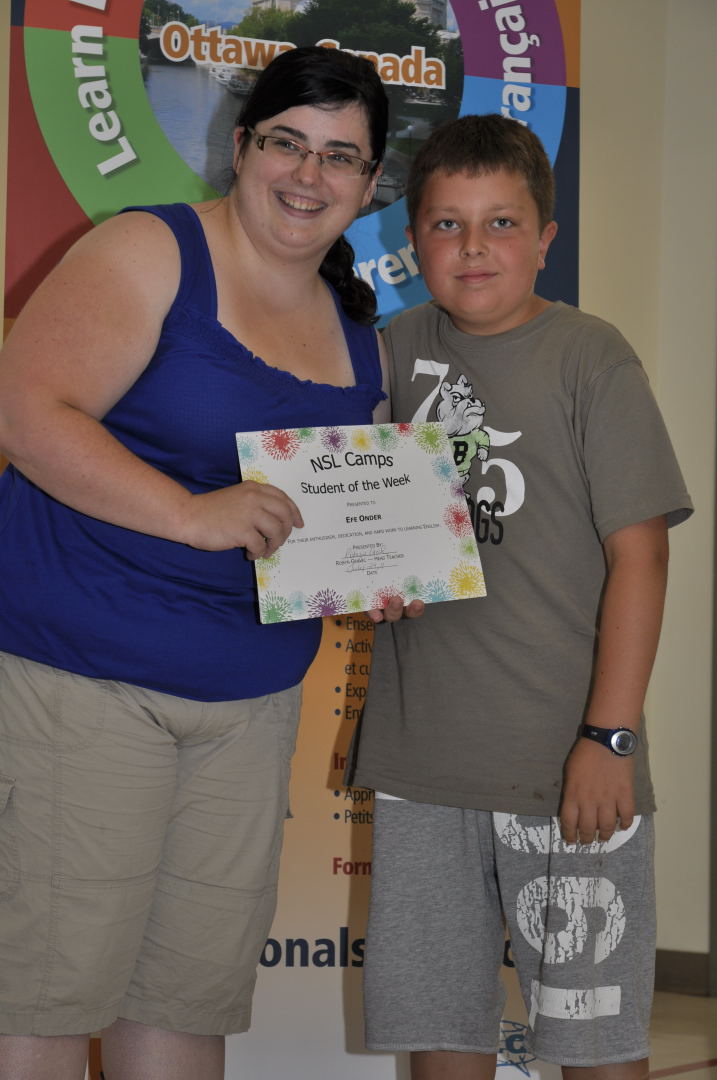In this vertical image, we see a woman and a young boy standing together. The woman, positioned on the left, has dark brown, almost black hair and wears glasses. She is dressed in a solid blue tank top with decorative elements like ruffles or lace at the top, and khaki cargo shorts. Beside her, the boy, who appears to be around 10 to 12 years old, almost matches her height. He is wearing a grey t-shirt featuring a bulldog and partial numbers "75," paired with grey cotton shorts adorned with part of the number "19" that stretches from the bottom up toward his knee. He accessorizes with a black watch on his left wrist, which has a silver display.

Both individuals are smiling and looking directly at the camera. The woman is leaning slightly towards the boy and holding an award certificate that features a colorful, firework-themed border. The text on the certificate reads "NSL Camps Student of the Week" with the name "Efe Onda."

Behind them, a colorful banner partially obscured by the woman's head displays the words "Ottawa, Canada" and "LEARN." To the right of the banner, a cream-colored wall or hallway is visible.